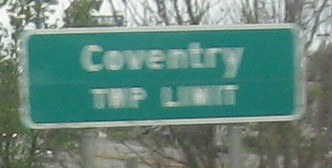The photograph captures a rectangular street sign with rounded corners, predominantly green with a white border. The sign prominently displays the word "Coventry" in white text, with an additional line below that is somewhat blurred and difficult to decipher, but it possibly reads "trip limit" or a similar phrase. The background features a dense array of tree branches and foliage, suggesting a verdant setting. Although the scene below the sign is somewhat ambiguous, there are hints of a roadway beneath, enhancing the impression of a leafy street or suburban area. The focus of the image remains tightly on the sign itself.